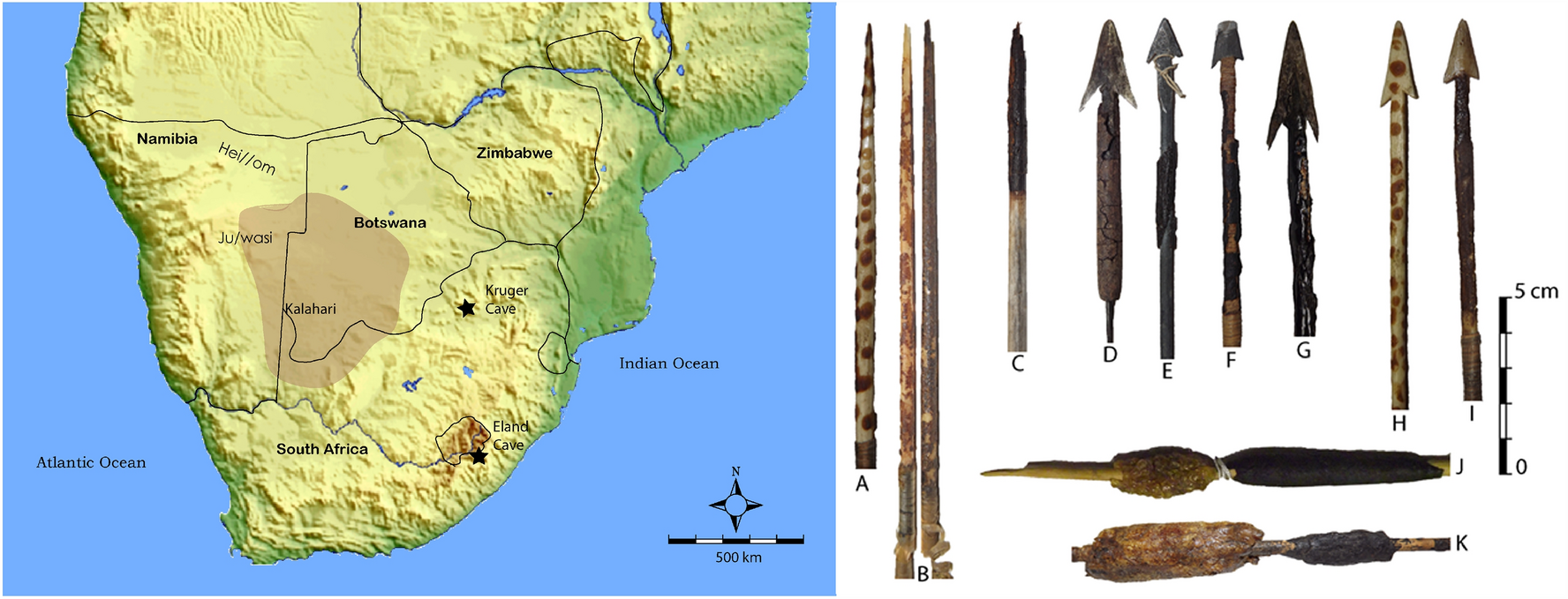The image is divided into two main sections. On the left side, there is a green and brown map of southern Africa, bordered by a yellow inner map and green outer edges, set against a blue background. The map highlights countries such as Namibia, Botswana, Zimbabwe, and northern South Africa, and also indicates the locations of the Atlantic and Indian Oceans. The brown areas on the map likely represent regions rich in metal resources. On the right side, there is a detailed diagram of various spears, labeled from A through O. These spears vary in color, including black, gray, off-white, and spotted red. The spears also differ in shape and design: some have pointed or rounded tips, while others are long poles. Below the standing spears are two cylindrical objects with distinct color variations, one featuring a dark left end with a brown circle and cylinder, and the other a combination of a brown oblong circle and a smaller black oblong with a stick protruding from it.